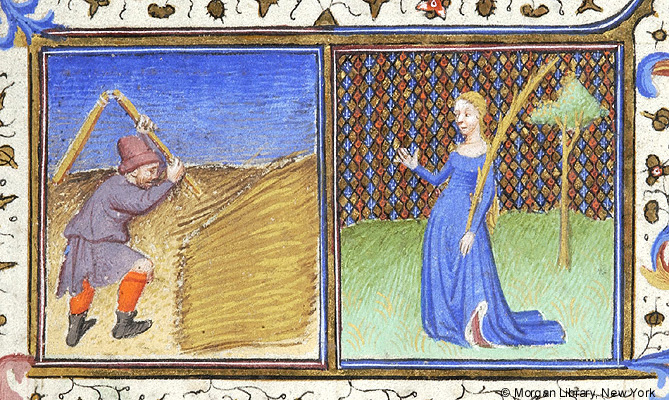The image features a pair of side-by-side illustrations originating from a medieval European manuscript. The artwork is encased in a brown decorative frame adorned with figures and scallops. The image on the left portrays a male peasant, set against a blue sky with a dirt ground. He wears black boots, red socks, a kilt-like skirt, a long-sleeved shirt, and a brown bucket hat. In his arms, he holds a sheaf of wheat high, appearing to thresh a nearby stack of golden wheat.

The right side of the image depicts a woman of possibly higher social standing, as indicated by her elegant blue gown. She stands in a meadow with green grass, a solitary tree beside her, and wears her long blonde hair braided down her back. She carries a large sheaf, similar to the one held by the man. Behind her stretches a tapestry-like background with diagonal shapes in brown, blue, and red. The border of the illustrations is richly ornamented with various patterns in a color scheme that mirrors the background. In the lower right corner, in small black font, reads the text "copyright Morgan Library, New York."